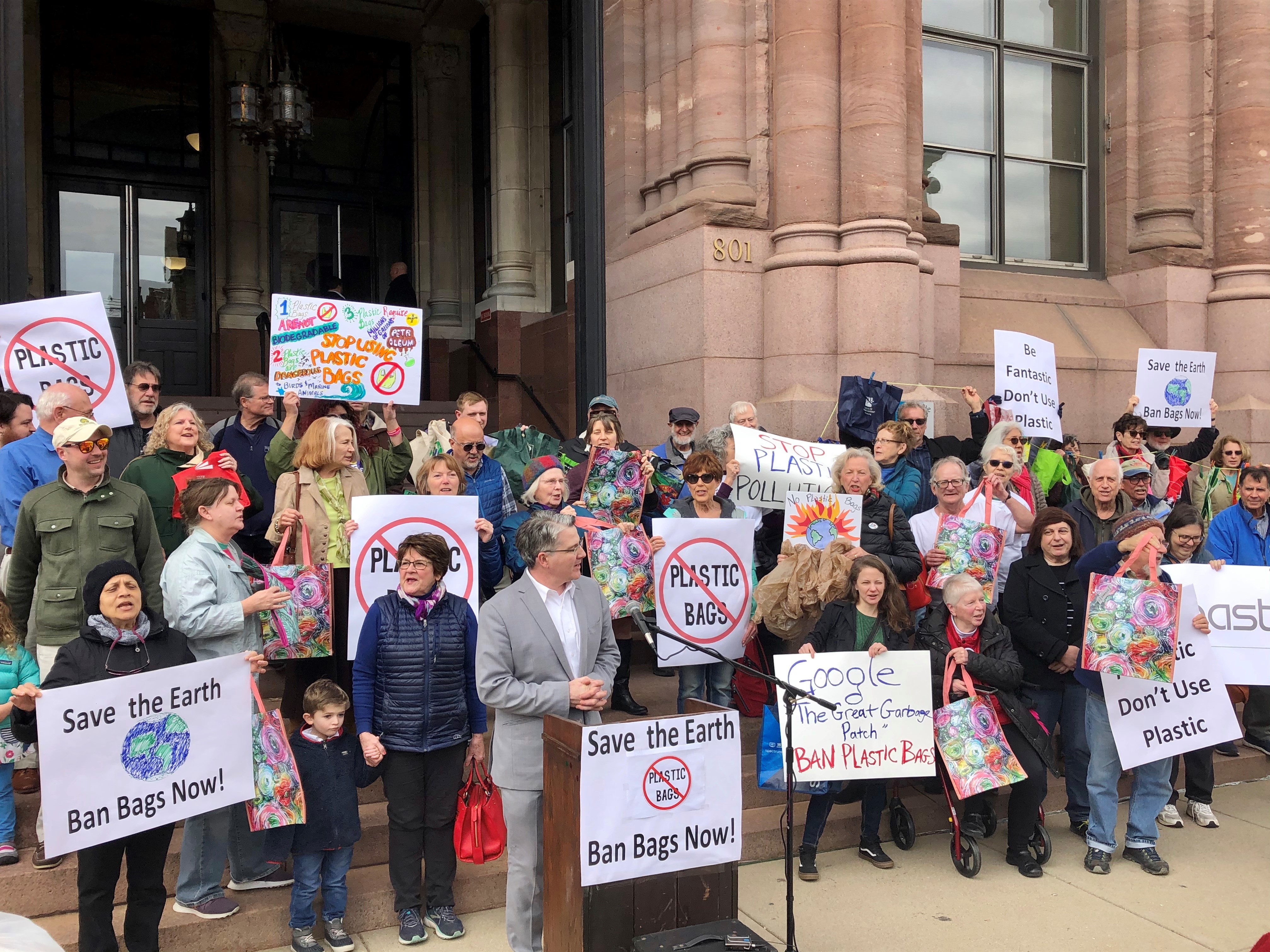The image is a color photograph of a protest taking place outside a large government building with stone columns, double entry doors, and a chandelier-type lantern hanging down in front. The scene features a diverse group of around 30 to 50 people, including children, adults, and elderly individuals, predominantly white with a few people of color. They are arranged on the steps and sidewalk in front of the building, bundled in heavy coats indicating a cold weather, possibly winter.

At the forefront of the gathering, a man in a suit stands at a podium inscribed with "Save the Earth, Ban Plastic Bags Now." He speaks into a microphone, appearing to lead the protest. Among the crowd, a woman in a wheelchair is seen alongside another woman standing next to her. The protesters hold a variety of handmade and printed signs with messages such as "Save the Earth, Ban Bags Now," "Ban Plastic Bags," "Don't Use Plastic," "Google the Great Garbage Patch," "Don't Be Fantastic, Don't Use Plastic," and "Stop Plastic Pollution," often featuring images like the Earth and plastic bags with red circles and slashes through them. The backdrop of the photo suggests an urban setting, possibly New York, with a brownstone style building.